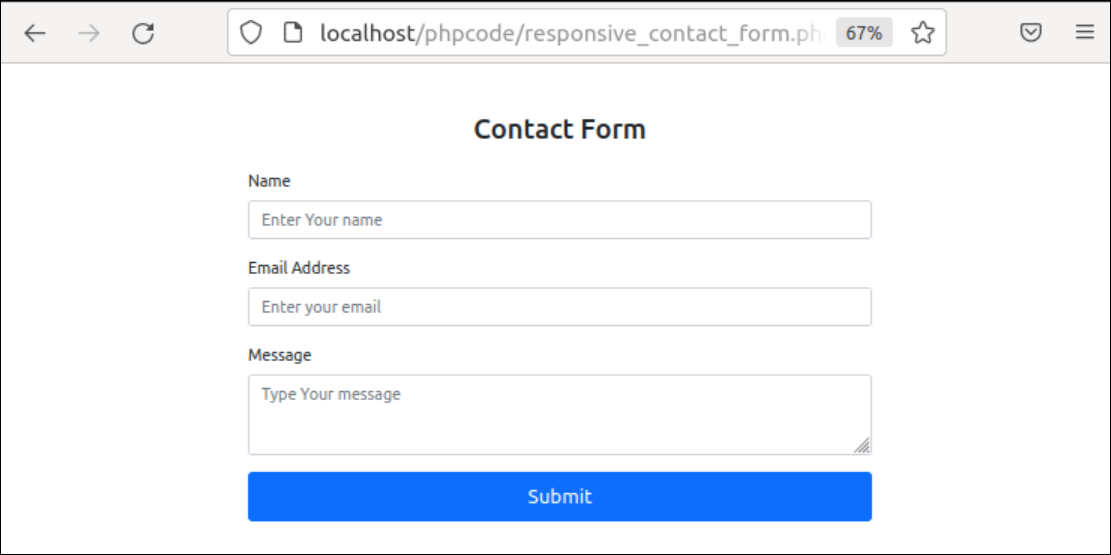The image is a screenshot of a webpage viewed on a browser, featuring a responsive contact form. Set against a white background, the browser interface includes navigational elements such as a left arrow, right arrow, and a refresh button. Notably, the right arrow appears in a gray color indicating an inactive state, while the other elements are in dark gray. The browser's address bar displays the URL: "localhost/phpcode/responsive_contact_form.php" and a zoom level of "67%". Additionally, the interface includes a star icon, a hamburger menu icon, and a badge with the letter "V", likely representing some form of verification or version information.

On the webpage itself, the central element is a contact form. The form fields include:
- "Name" with a placeholder "Enter your name"
- "Email Address" with a placeholder "Enter your email"
- "Message" with a placeholder "Type your message"

Below these fields, there is a blue rectangle containing an arrow, which functions as the submit button. Additionally, there is another button labeled "Wipe" for clearing the form. The design and layout of the form are clear and user-friendly, emphasizing ease of use for contacting the website's administrators or support team.